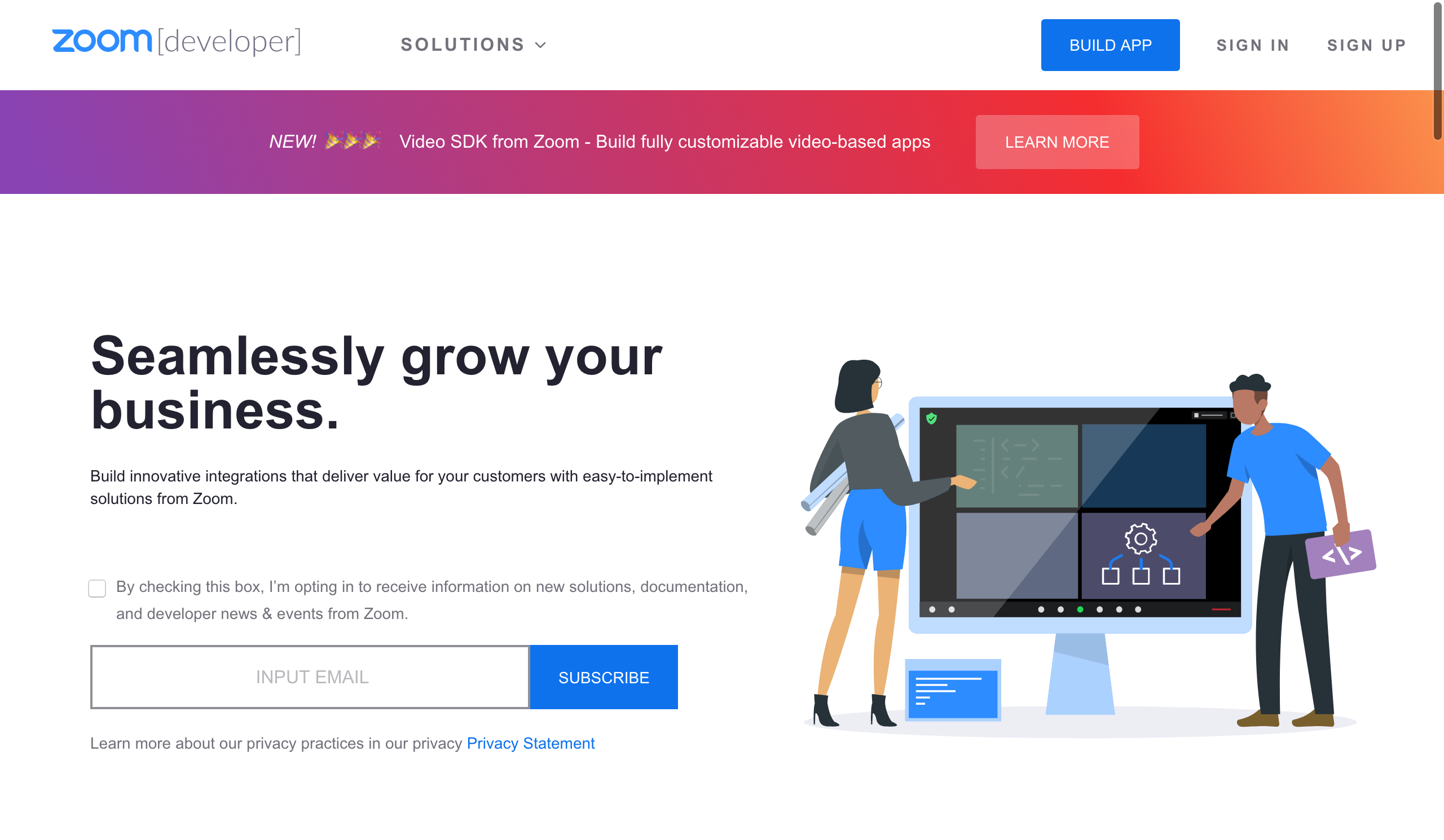### Caption:

The website for the business Zoom features a sleek and informative layout. At the very top, "ZOOM" is prominently displayed in all capital blue letters. Next to it, in small lowercase within parentheses, it reads "developer."

Below the header, there is a navigation tab labeled "Solutions" with a downward arrow, indicating a dropdown menu for more options. On the right-hand side of the header, a blue rectangle with white letters says "Build App," flanked by "Sign In" and "Sign Up" options.

Beneath this primary nav bar, a gradient box transitions from purple on the left to red on the right. It contains the word "NEW!" in all caps followed by three party-horn emojis. Next to this eye-catching announcement is a description of Zoom’s latest feature: "Video SDK from Zoom - Build fully customizable video-based apps." A "Learn More" button is provided for additional information.

Dominating the center of the page, a bold black headline declares, "Seamlessly grow your business." Below, in smaller text, the site elaborates, "Build innovative integrations that deliver value for your customers with easy to implement solutions from Zoom."

To the right of this central text, a graphic featuring cartoon figures adds a creative touch: a woman in blue attire with a short braid, wearing a long-sleeved shirt and black booties, holds rolled-up business graphs and charts under her arm as she gazes at a large TV screen. Beside her, a man dressed in a blue t-shirt and black pants points towards the TV, emphasizing collaboration and strategic planning.